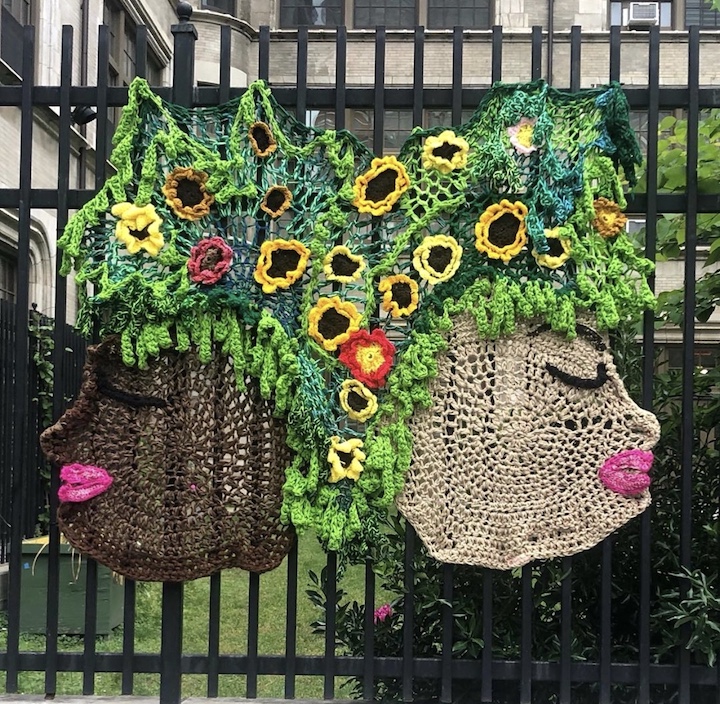This image captures a piece of intricate, handmade yarn art suspended on the upper part of a black wrought iron fence. The fence, characterized by its vertical and horizontal metal bars, provides a dramatic contrast to the colorful artwork. The knitted piece features two human faces: one representing a darker-skinned individual and the other a lighter-skinned individual, both adorned with prominent pink lips and eyes that appear to be closed, crafted from black yarn. Their interconnected hair is a vibrant tapestry of green yarn strands woven with various flowers, including yellow sunflowers, orange blooms, and a single red flower, giving a net-like appearance. Behind the fence, partially visible, is a beige building with windows and an air conditioning unit, suggesting it might be an apartment complex. In the bottom right corner, bushes and grassy areas add a touch of natural greenery to the scene, blending seamlessly with the artistic depiction on the fence.